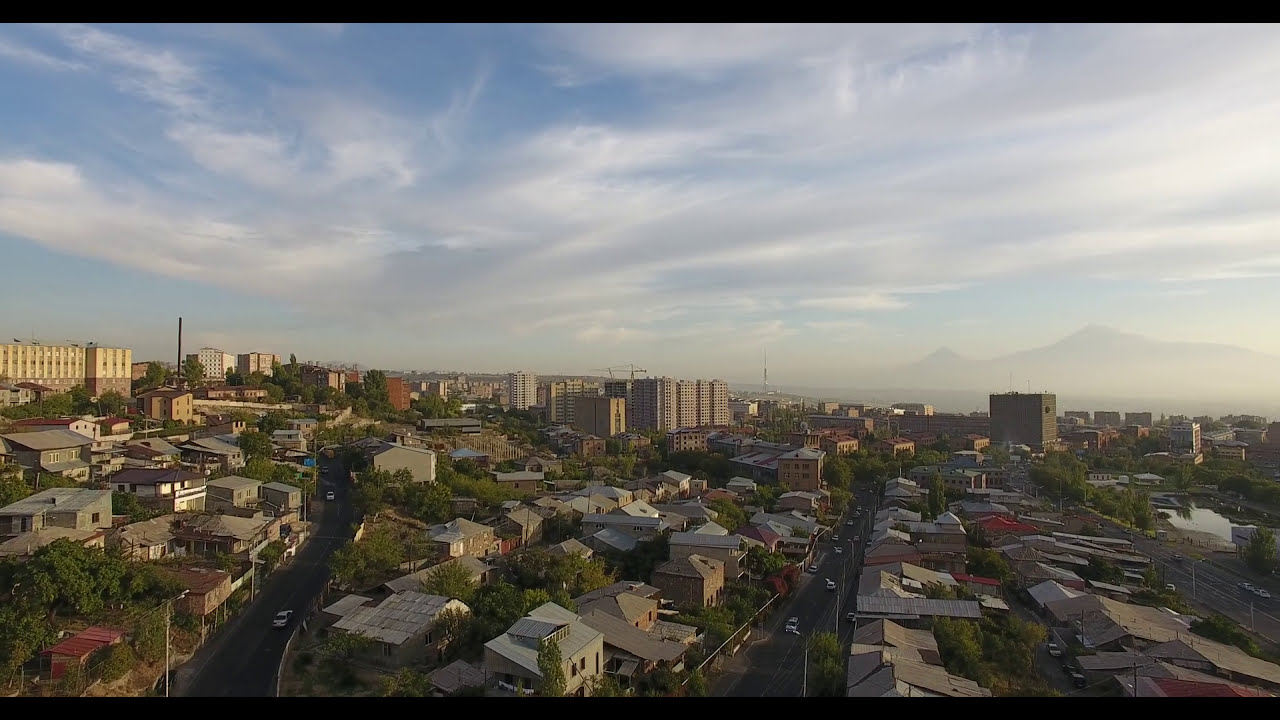This is an aerial photograph capturing a sprawling city scene from an elevated vantage point. The foreground of the image features a neighborhood with a variety of houses in shades of white, brown, beige, and red, interspersed with lush green trees. Three parallel roads weave through this area, populated by numerous moving vehicles. As the eye moves further back, the urban landscape transitions from these lower buildings to an array of towering high-rises. These tall structures are primarily gray and brown, with a prominent red building adding a striking contrast. The sky, which occupies about half the photograph, is a vibrant blue adorned with white streaky clouds, suggestive of an early morning glow. The sun’s rays illuminate the buildings, highlighting their details and casting a clear natural light over the entire scene. In the distant background, blurry with fog, the silhouette of mountains and hills adds depth to the composition, seamlessly blending natural and urban elements.